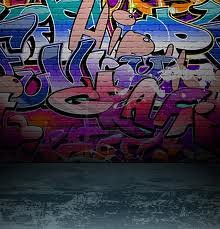This photograph captures an outdoor brick wall adorned with vibrant, intricate graffiti, situated in what appears to be an urban environment. The graffiti is exceptionally colorful, featuring hues of bright pink, teal, dark blue, indigo, white, yellow, green, and orange. Despite the vivid colors, the text is highly stylized and chaotic, making it difficult to decipher specific words or messages. A notable section appears to spell "hip" in pink, while another portion suggests the word "graffiti," though some letters are obscured or cut off. The wall's brick texture is visible beneath the layers of spray paint, adding depth and dimension to the artwork. The ground in front of the wall seems to be asphalt or concrete, possibly painted but worn, and has a greenish tint in some areas. The photograph possibly captures an evening or interior setting, indicated by an artificial light source illuminating the scene, adding to the artistic ambiance of this urban tableau.